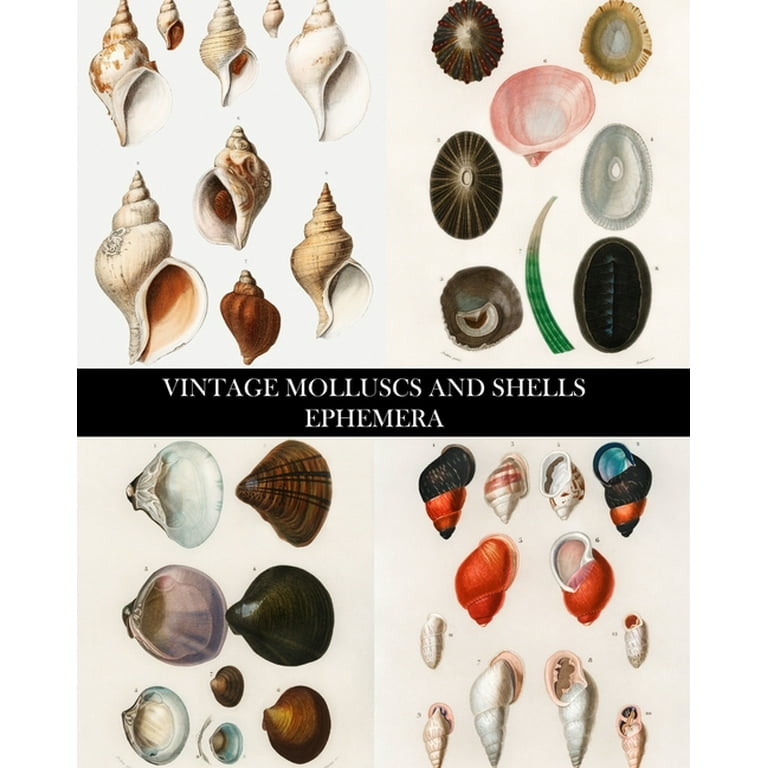The image showcases the front cover of a book featuring an array of differently shaped mollusks and shells, titled "Vintage Mollusks and Shells" with the word "Ephemera" beneath it, both inscribed in white text on a black band across the center. The cover is divided into four symmetric sections, each displaying a collection of shells grouped by similarity. The upper sections exhibit rounder shells and conch shells, while the lower sections showcase smaller, cone-shaped shells on the left and clam-like, pearl-containing shells on the right. The overall color palette includes shades of orange, black, green, light pink, white, brown, blue, light blue, and beige, with light brown and other earthy tones being predominant. The detailed arrangement and vintage aesthetic suggest a comprehensive guide to mollusks and shells.